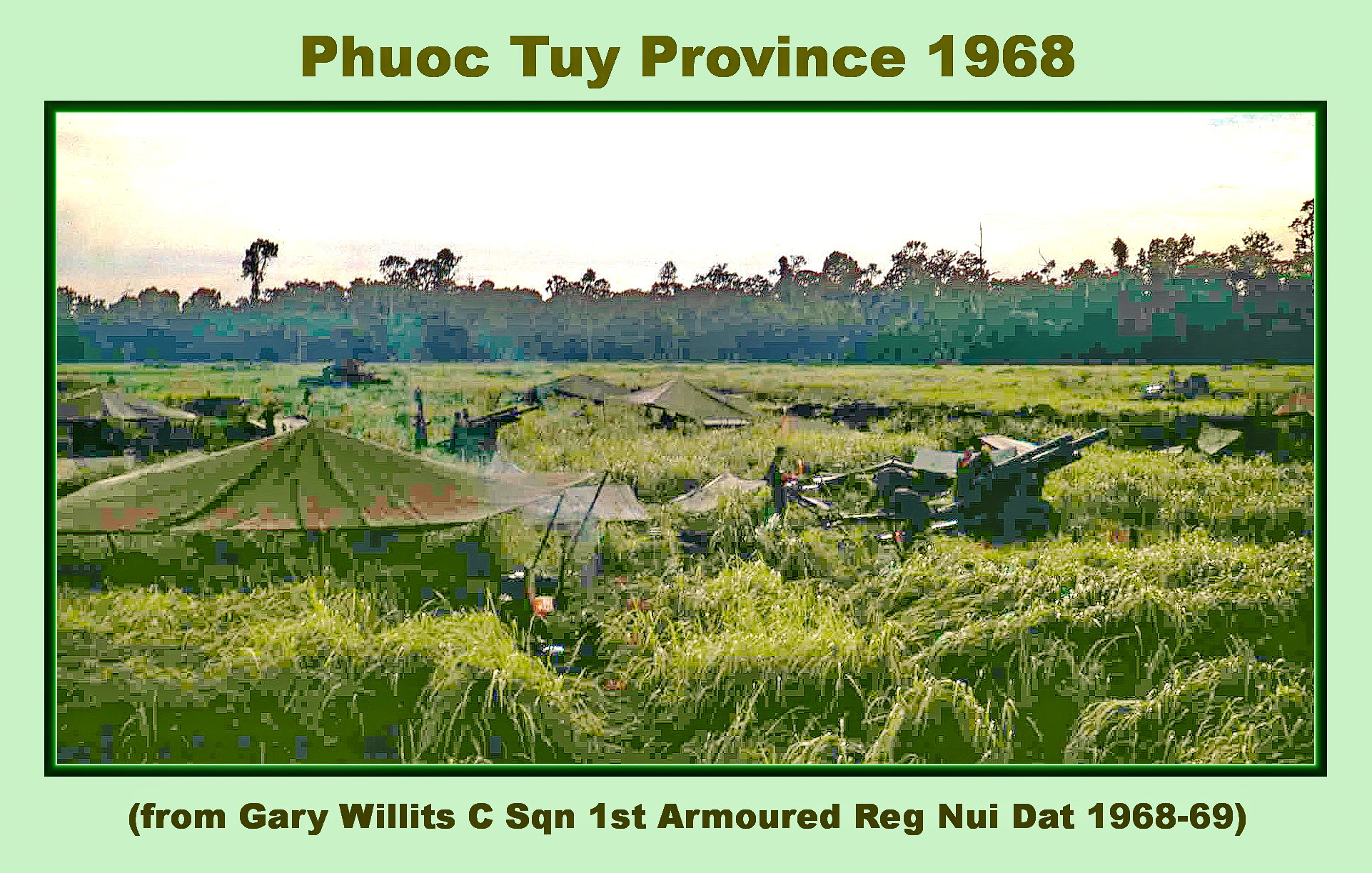This detailed image postcard, titled "Phuoc Tuy Province, 1968," originates from Gary Wilkes' (often misspelled as Gary Willett or Willis) Captain's Squadron, 1st Armored Regiment, covering their activities from 1968-1969 during the Vietnam War. The scene is set in a military encampment located in a high grass, open field encircled by dense woods. Soldiers are seen operating machine guns and artillery, giving insight into their daily operations. The area appears clean, with no immediate signs of conflict, and the air is thick and humid, indicating typical tropical conditions. In the background, tall trees are visible under a cloudy sky. The image quality is notably poor, with significant pixelation and digital artifacts, including blue squares and a green hue possibly due to digitization or age. The soldiers are partially obscured by camouflage netting, adding to the overall military ambiance of the postcard.